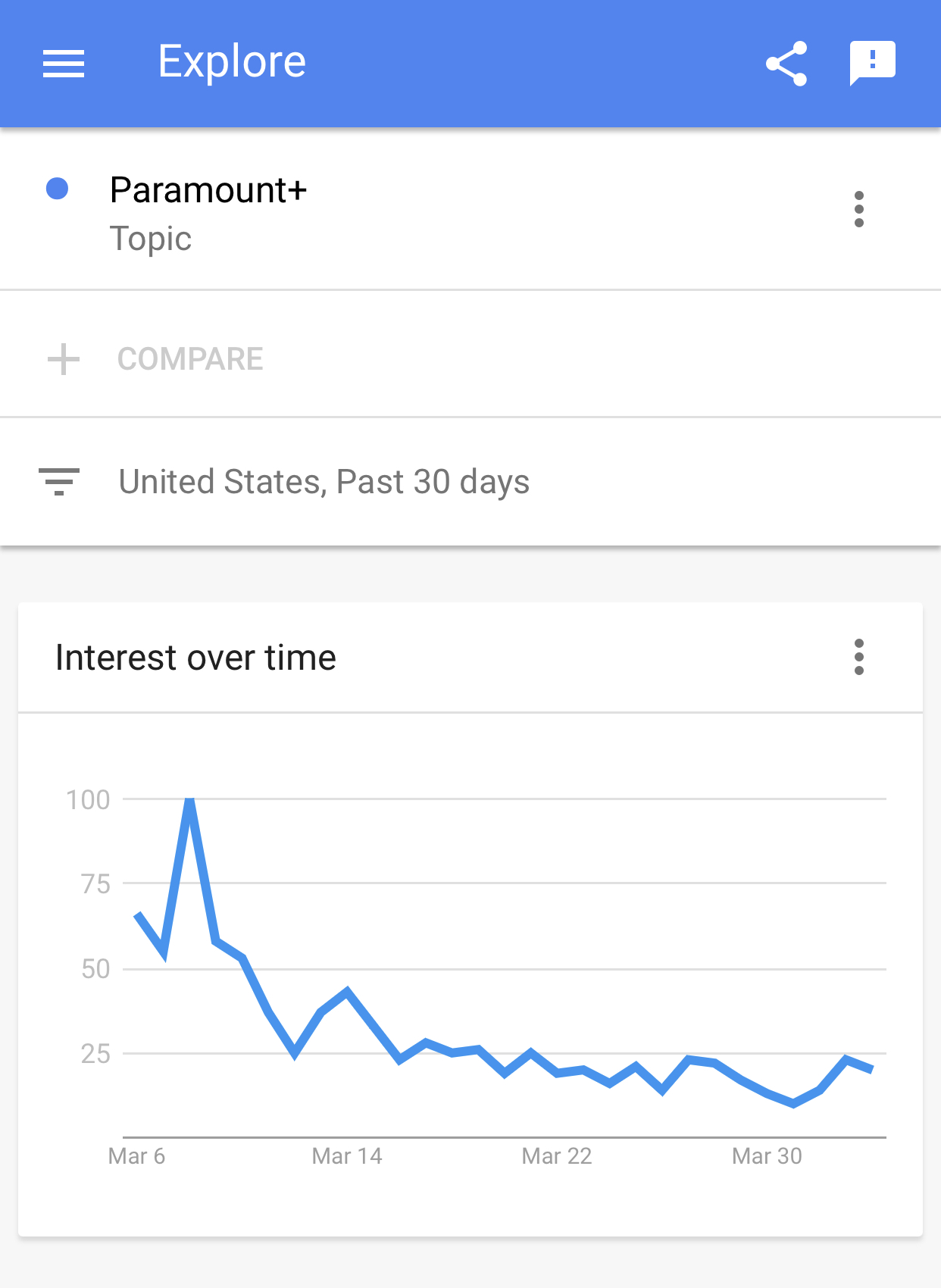This image showcases a screenshot from a website, likely captured on a Samsung Galaxy tablet. At the top of the screenshot, there's a wide blue banner. On the left side of this banner, there's a three-line hamburger menu icon, followed by the word "Explore" to its right. Towards the far-right side of the banner, there are three more icons: a share icon, a square comment icon with a blue-highlighted quotation mark inside.

Beneath the banner, on the left side, a blue dot precedes the text "Paramount Plus." Right below this, the word "Topic" appears in light gray. On the right side, there are three vertical dots. A horizontal line separates this section from the following content.

Next, the word "Compare" is displayed with a plus sign to its left, leading into another horizontal line. Below this line, three bars of varying lengths (small to large) are arranged horizontally. The text "United States, past 30 days" follows these bars, and beneath this, there's a gray-shaded area.

A box labeled "Interest Over Time" is positioned below the gray space, presenting data from March 6th to March 30th. The chart starts at a point between 70 and then declines to below 25.